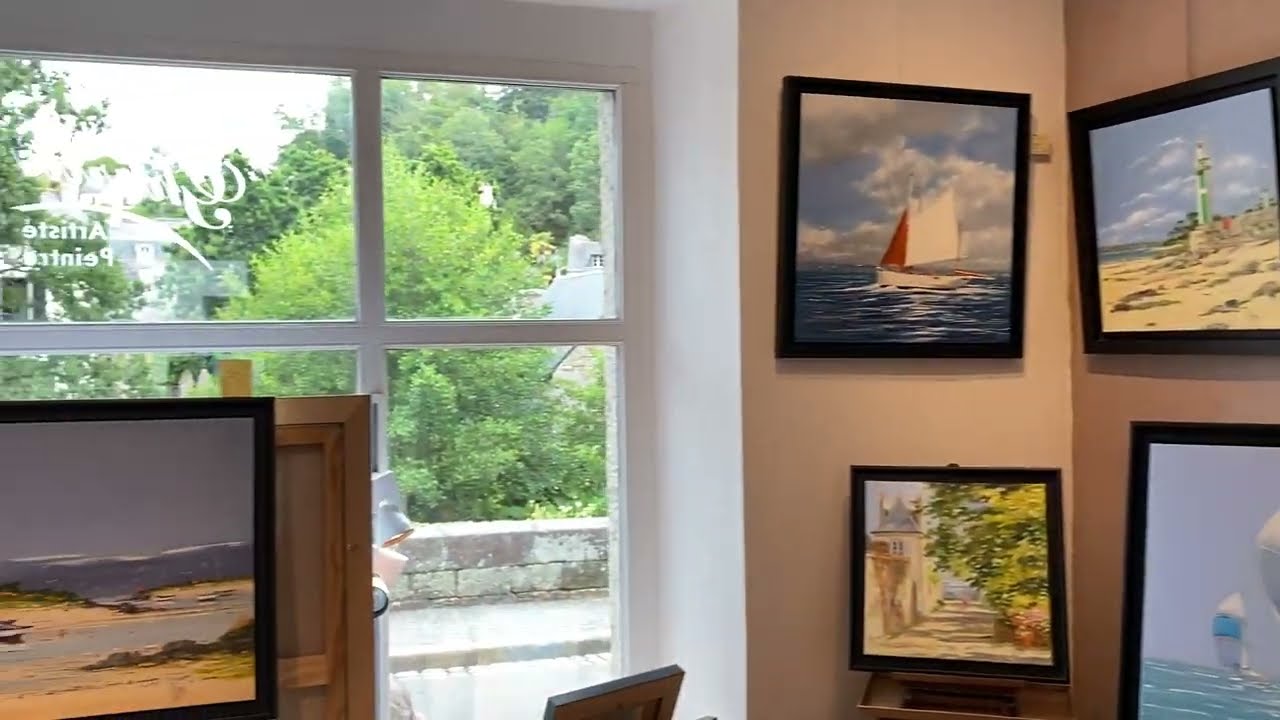The photograph captures an indoor setting of an art gallery or art store during the daytime. Dominating the scene on the left is a large window with writing on it, possibly in a different language, including the word "artiste." The window reveals a view outside to a low stone wall and green trees. On the right side of the image, beige walls are adorned with at least five framed pictures, each depicting serene outdoor scenes, mostly involving water. One picture shows a ship on the water, another features a lighthouse near the shore, while others depict a city path and multiple beach scenes. The frames are all black, with one noticeable picture in a black frame positioned at the bottom left near the window, showcasing a beach scene. The overall color palette includes white, beige, brown, red, blue, light blue, gray, yellow, light green, and dark green.